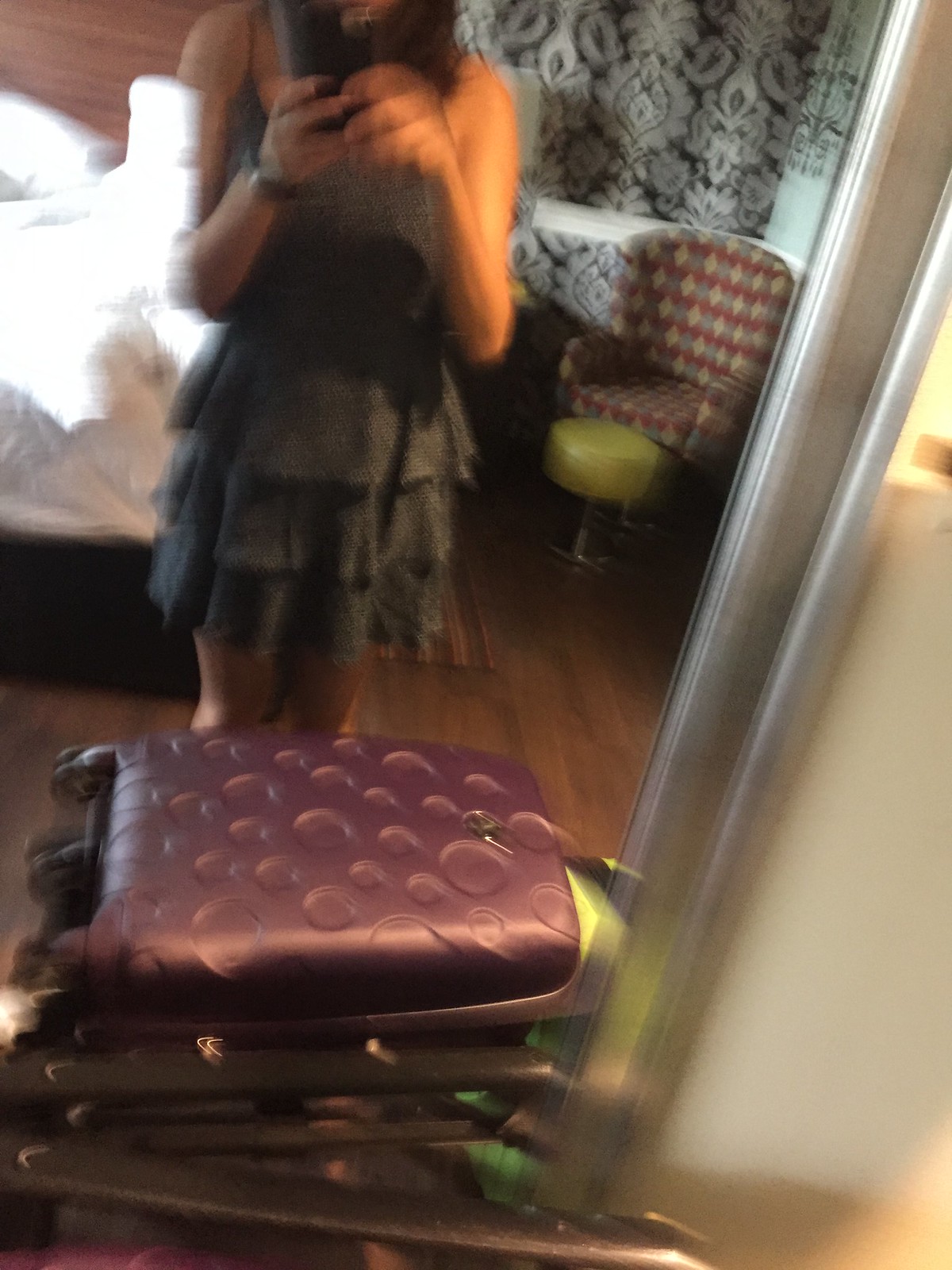This photograph captures a blurry image of a woman in a black dress taking a selfie in front of a large mirror using her phone. The mirror occupies the entire left side of the photo, stretching from the bottom middle to the top right corner. The woman is positioned in the top left area of the reflection, with both hands holding the black phone in front of her chest and face. Her black dress features a flowy design around the waist. 

In the foreground, at the bottom left, a purple suitcase with black wheels lies on its back. The room's flooring is a dark brown wood, complementing the black and white floral wallpaper that adorns the wall behind her. Nearby, an argyle-patterned chair sits with a yellow stool positioned in front of it. To the left of the image, there is a white bed covered with a white sheet.